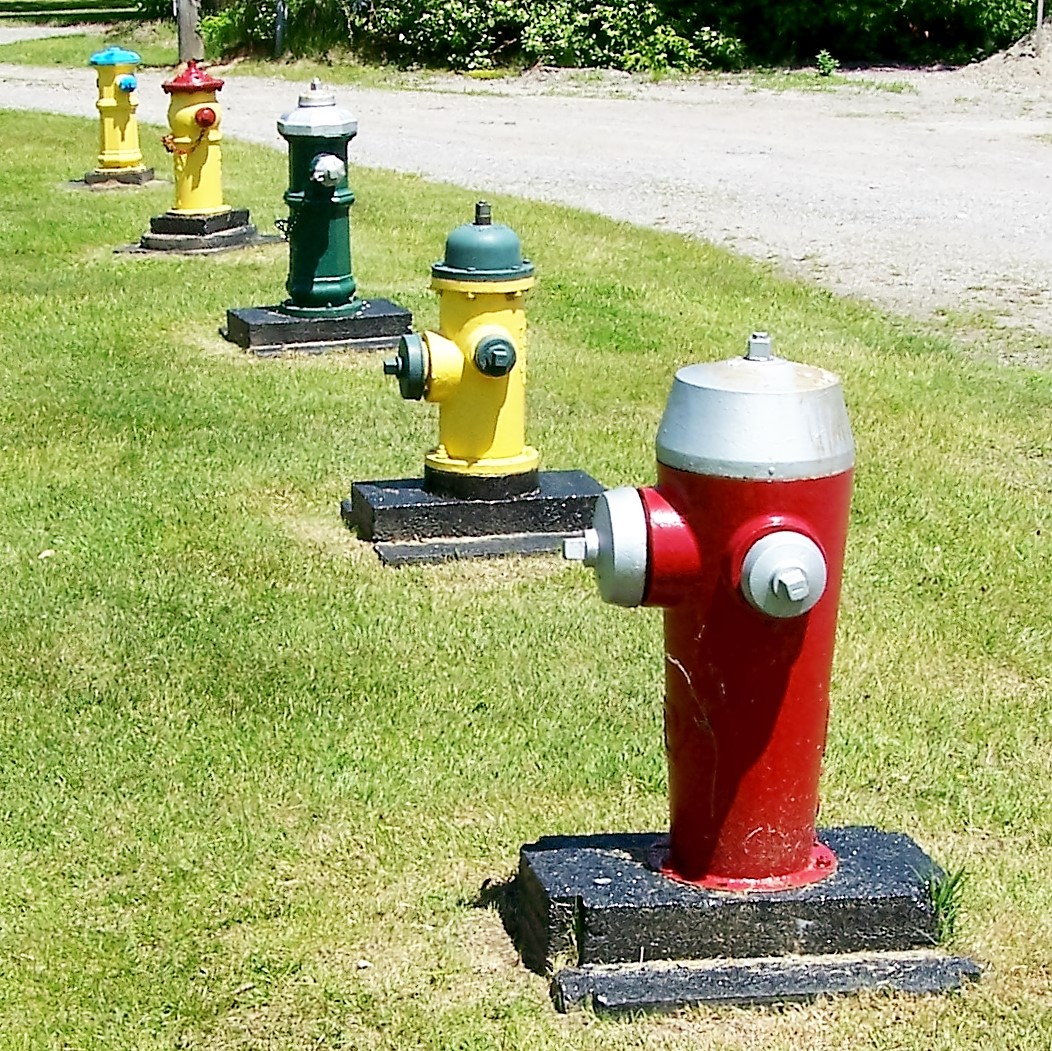In this daytime photograph, we see a square image featuring a vibrant green lawn, beyond which a dirt road runs diagonally across the frame. Situated on the lawn are five fire hydrants lined up in a row, each positioned on a black concrete platform. Starting from the bottom right, the first fire hydrant is predominantly red with a white top. The second hydrant is yellow with an army green top. The third one is dark green with a silver top. Moving further back, the fourth hydrant is yellow with a red top. Slightly to the left and further behind, the fifth hydrant is yellow with a bright blue top. The dirt road creates a natural border that accentuates the orderly arrangement of the hydrants on the lush green grass.